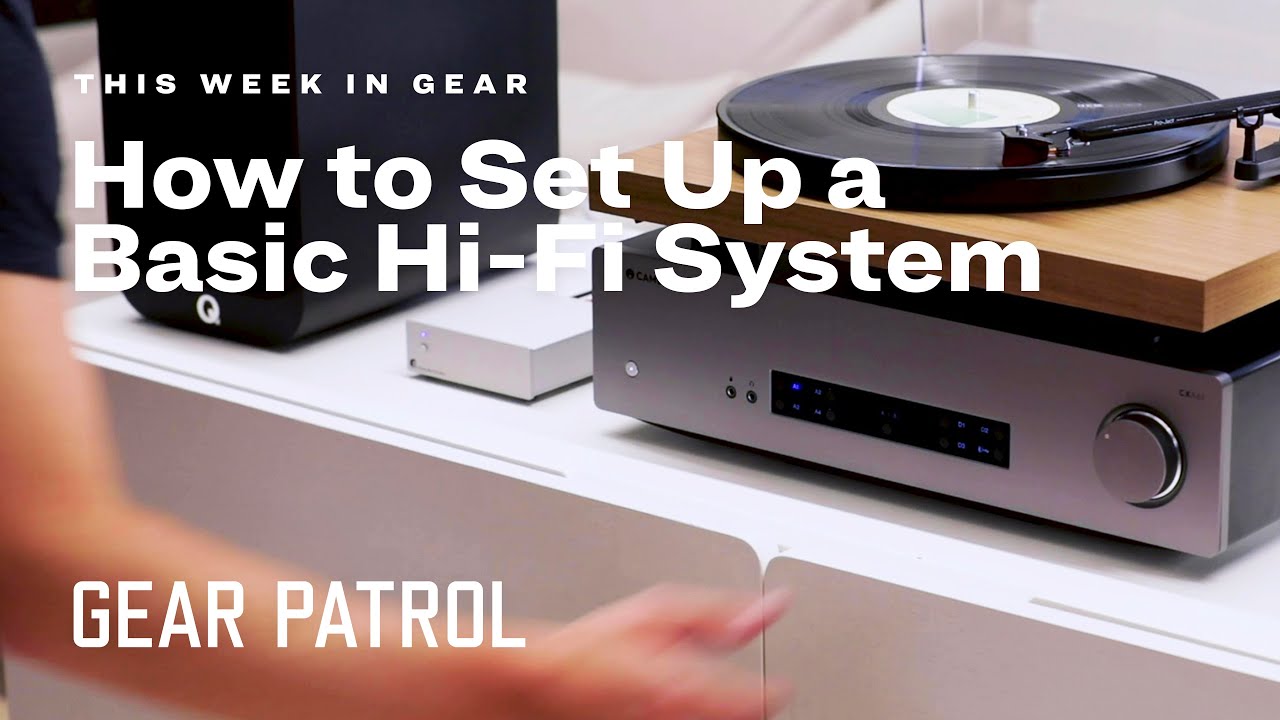The image is a rectangular advertisement that is wider than it is tall with a primary focus on setting up a basic hi-fi system. The advertisement's text is displayed in white, stating "This Week in Gear, How to Set Up a Basic Hi-Fi System," with "Gear Patrol" written at the bottom left corner. The main photograph showcases a modern turntable with a metallic silver or gray base and a wooden-colored top, positioned on a white shelf. The turntable holds a record with the needle poised as if playing music. To the right of the turntable is a small white box and a black component resembling a computer base or additional audio equipment. The scene also includes a blurred arm, presumably of a woman, reaching out towards the turntable, possibly to adjust the volume or interact with the system in some way.